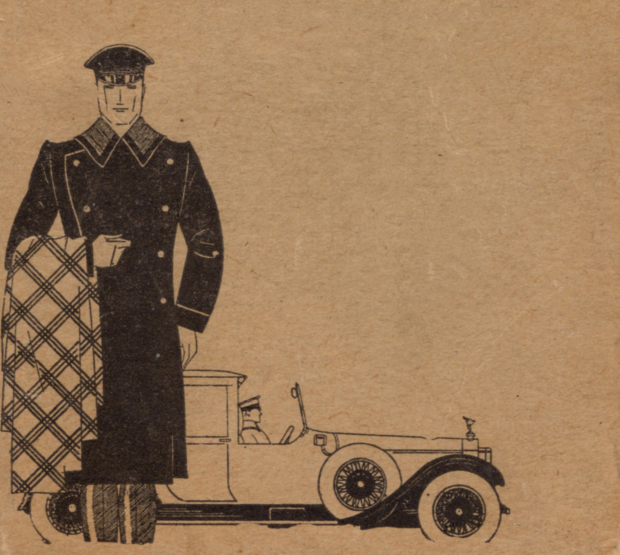The black-and-white ink drawing captures a nostalgic scene from the early 1930s, featuring an old-fashioned Ford car. Central to the image is a man, likely a chauffeur, standing confidently in front of the car. He is dressed in a long, black trench coat with eight prominent buttons and two large collars. His attire is completed with a black driver's hat and striped slacks. Held in his right hand is a plaid-patterned towel. Behind him, a second driver is visible, seated in the car and wearing a white uniform and milkman-style hat. The Ford, facing to the right, is detailed with classic features including a central hood ornament, white tires, and black-accented rims. The background, suggestive of a wall with flecks and cracks, adds to the vintage ambiance of the scene.